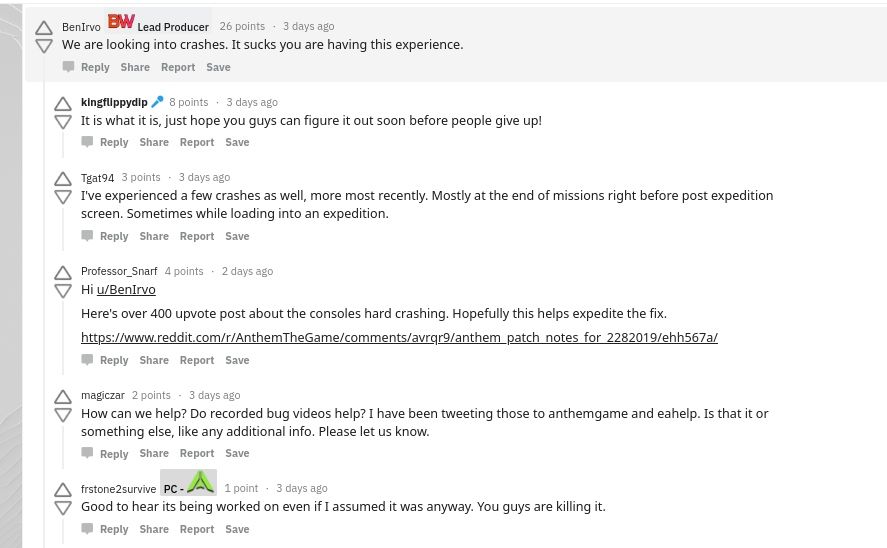**Screenshot of a Reddit Thread Discussion on Game Crashes**

This image captures a detailed Reddit thread discussing crashes in a popular game. The top comment, posted by Ben Ervo, the lead producer, has accumulated 26 points within three days. Ben acknowledges the crash issues, stating, "We are looking into crashes. It sucks you are having this experience."

A user named King Flippy Dip replies, "It is what it is. Just hope you guys can figure it out soon before people give up."

The thread continues with various comments:

1. **User Tooka_94:** "I've experienced a few crashes as well, mostly at the end of missions right before the post-expedition screen, and sometimes while loading into an expedition."
   
2. **Professor Snarf:** "Hi Ben Ervo, here's an over 400 upvotes post about the consoles hard crashing. Hopefully, this helps expedite the fix." (The post includes a link to the Anthem subreddit.)

3. **Magic Czar:** "How can we help? Do recorded bug videos help? I've been tweeting those to the Anthem game and EA Help. Is there anything else, like any additional info, you need? Please let us know."

4. **Final Comment:** "Good to hear it's being worked on, even if I assumed it was anyway. You guys are killing it."

These replies directly address Ben Ervo's comment, reflecting a community eager for solutions and willing to assist in troubleshooting the game.